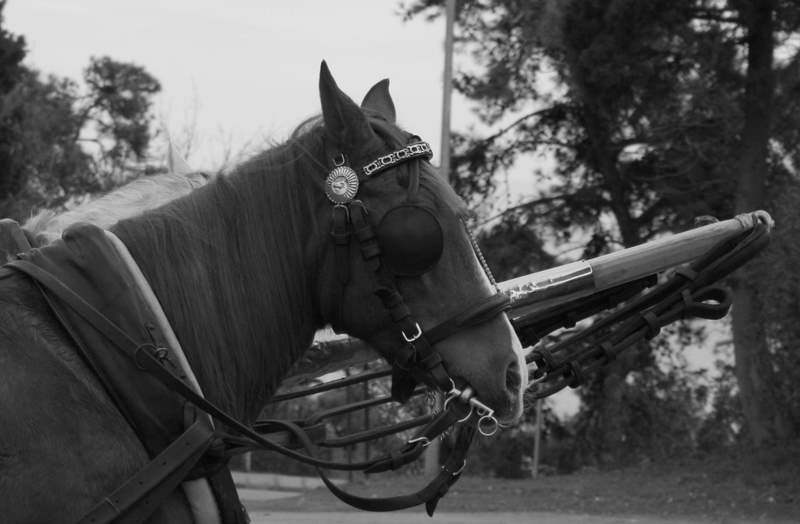In this wide-angled black and white photograph, a well-groomed horse is prominently featured as the central subject. The horse, dark in hue with a smooth mane and a white stripe down its face, is adorned with an eyepatch over its right eye and a headband with designs. It is also equipped with blinders, reins, and other carriage apparatus, indicating it is likely part of a horse and carriage setup. The background reveals a smattering of somewhat indistinct conifer trees, suggesting a sparse forest setting. The horse appears to be patiently waiting, possibly ready to pull a carriage, with another barely visible white horse suggesting it could be part of a pair. The composition of the photograph artfully centers the horse's head, capturing both its calm demeanor and readiness for action.